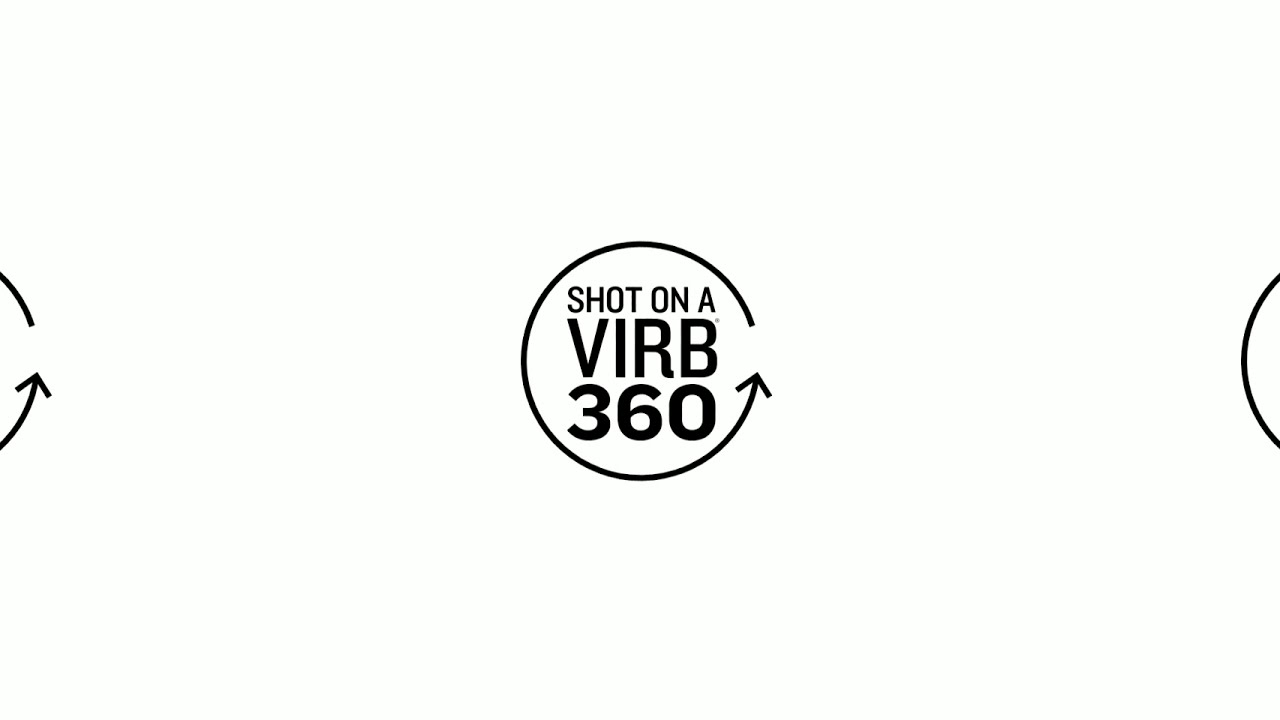The image is a computer-generated minimalist logo for a 360-degree camera, prominently featuring a circular arrow design. In the center of the circle, the text "shot on a" is placed on one line, followed by "VIRB" in much larger, bold lettering on the next line, and "360" in even larger, bolder lettering below. The arrow completes almost a full circle around this text before ending at the arrowhead. The logo is displayed on a white rectangular background, with the circular arrow and text in black. The image appears cropped, with parts of the circular design repeating on both the left and right edges of the frame. The logo effectively conveys the notion of a 360-degree camera shot, likely signifying the branding for a digital camera product.